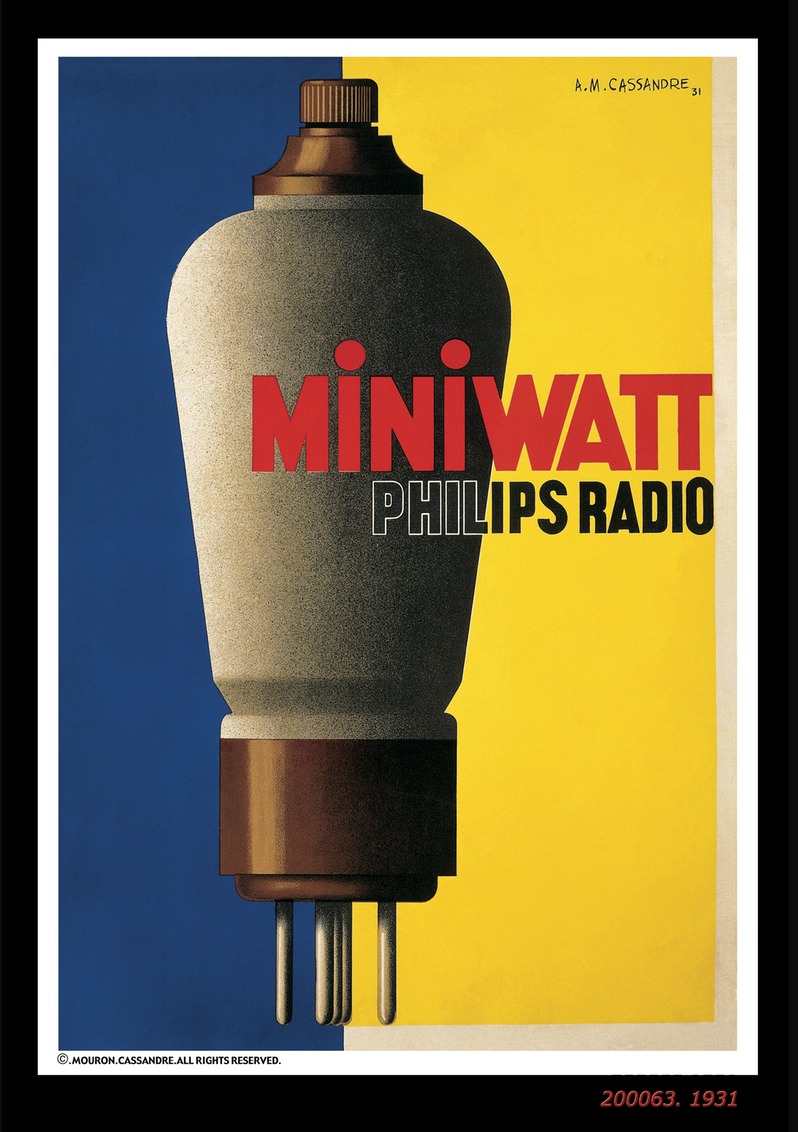This is an advertisement poster for Philips Radio, featuring a stylized illustration of a plug-in device resembling a vintage, vase-shaped bulb with a metallic brown base and four prongs. The bulb appears to be made of a grayish concrete-like material, with the top section copper-colored with a twist knob. The design is set against a dual-colored background: blue on the left and yellow on the right. The centerpiece of the poster is prominently marked with "MINIWATT" in bold red letters, with "Philips Radio" written in black below it. The poster is signed by A.M. Cassandre in the top right corner, with the year '31, signifying 1931. The bottom left corner notes the copyright information "©Mouron Cassandre, All Rights Reserved," while the lower right corner features the text "200063.1931" in red or rust-colored orange. The entire poster is bordered in black, with an inner white margin.